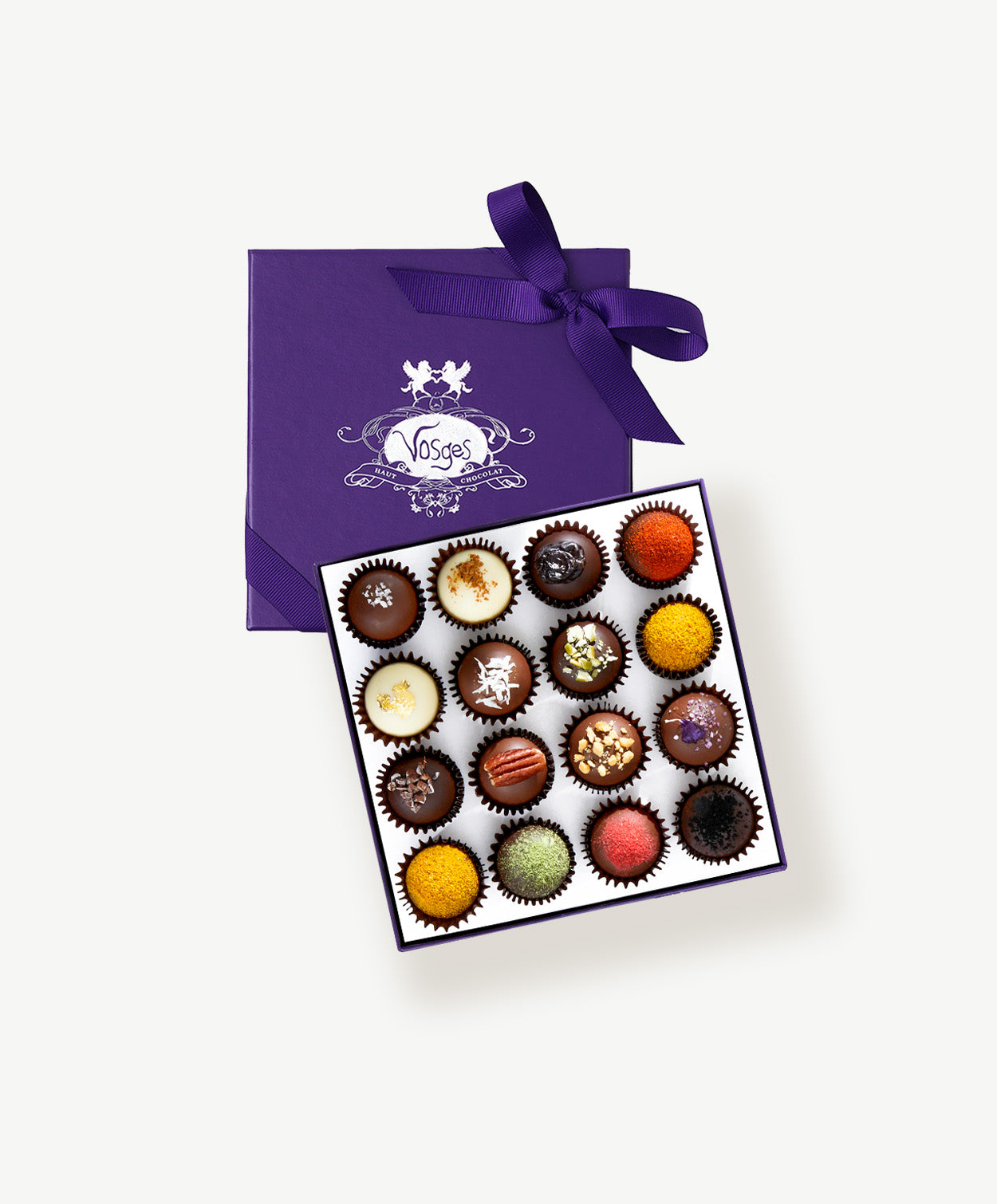This image showcases an elegant arrangement of 16 assorted chocolates displayed in a luxurious gift box, photographed from a top-down perspective against a white background. The box itself is black with a white interior, and each chocolate is neatly nestled in individual white compartments set in four rows and four columns. 

The box lid, tucked beneath and angled slightly to the left, is a rich dark purple adorned with a satin bow in the upper right corner. At the center of the lid, the brand name 'Vosges' (V-O-S-G-E-S) is prominently displayed in white lettering within an ornate oval design featuring two winged horses facing each other.

Each of the spherical chocolates varies in flavor and decoration, presenting a delightful array of colors and textures. Some chocolates are dark brown with black accents, others are white with brown or colorful toppings, including vibrant hues like orange, yellow, green, and red. Nuts such as pecans and peanuts, as well as coatings like coconut flakes and colored powders, add to the intricate detailing of each piece. The harmonious blend of colors and designs contributes to the overall visual appeal, making the assortment look incredibly appetizing and luxurious.